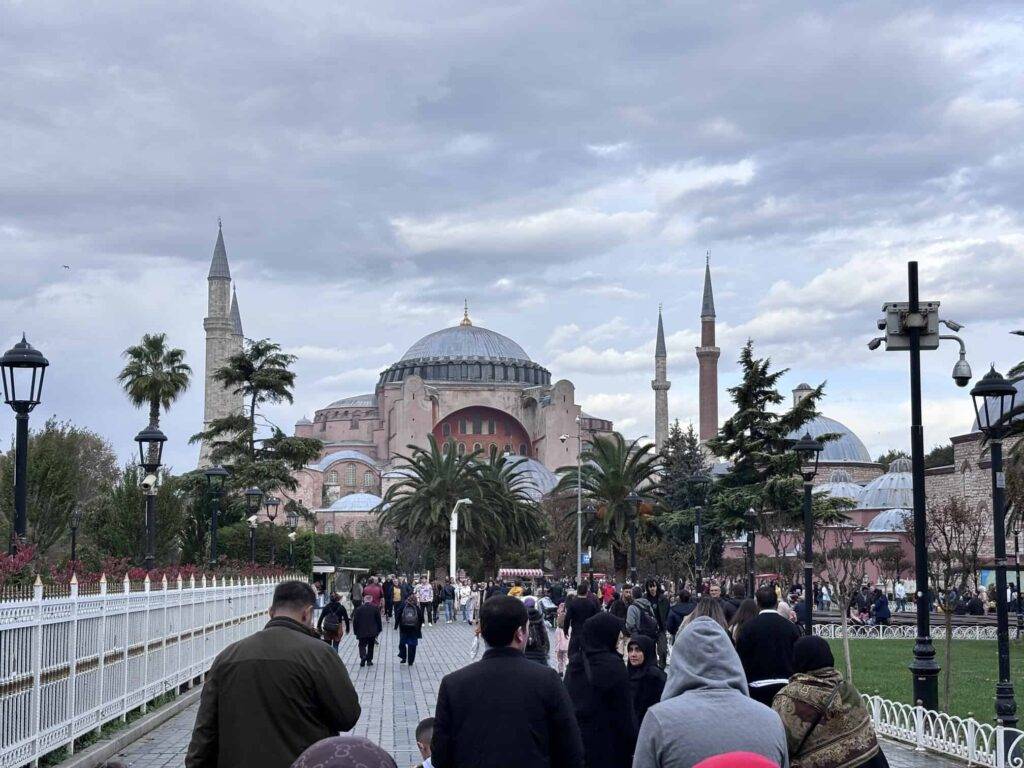The image depicts a bustling scene of visitors making their way along a brick-paved pathway towards a grand monument, reminiscent of a mosque with features similar to the Taj Mahal. Dominating the upper half of the picture is a mostly cloudy sky, with scant patches of blue closer to land on the right. The imposing structure in the background features a large central dome, a prominent spire, and several slender, spindly towers that echo the architectural style of minarets. The pathway leading to this magnificent edifice is flanked by palm trees, a white painted wrought iron fence, and street posts on either side, enhancing the regal ambiance of the approach. A green lawn borders the walkway, further adding to the scenic view. The visitors, seen from behind, are dressed in coats and hoods, indicative of cooler weather, and their presence adds a lively human element to this serene yet grand setting.